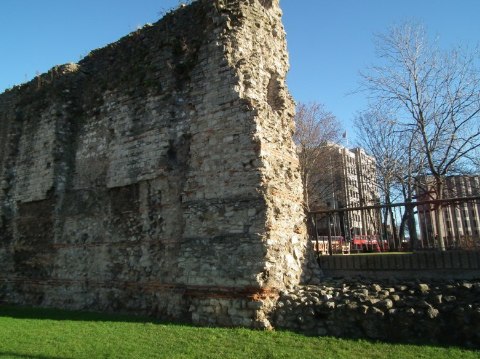The photograph depicts a towering, ancient stone wall to the left, appearing worn and weathered with numerous gray and black patches, and adorned with darker green ivy at the top. The wall, roughly 20 feet high and 4 inches thick, has a rugged, jagged edge, as if split in half. Below the wall lies a short, green grassy area, and a rock pathway extends to the right. In the distant background, one can see modern high-rise buildings standing behind bare trees, all set against a clear blue sky. The remnants of this deteriorated wall evoke a sense of history, perhaps once serving as a protective barrier for an old castle or village.